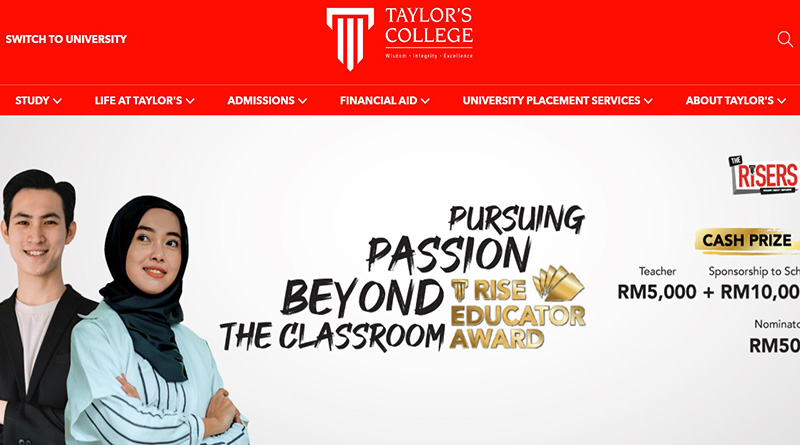In the image, the top portion prominently displays the text "Taylors College" in bold white letters, set against a deep red background, indicating that the page pertains to Taylors College. To the left of the text is the Taylors icon, featuring a stylized 'T' formed by three vertical lines with a white line across the top. On the far left, there's an option labeled "Switch to University."

Below this header are six tabs or drop-down menus: "Study," "Life at Taylors," "Admissions," "Financial Aid," "University Placement Services," and "About Taylors," all written in white against the red background. On the right side of this header, you'll find a white search bar.

The main body of the page has a clean white background. Dominating the central part of the page is a bold black text that reads, "Pursuing Passion Beyond the Classroom." To the right of this text, "RISE Educator Award" is displayed in a striking gold font. Further to the right are the details of the RISE Awards: "The RISER's Cash Prize Teacher: RM5000," "Sponsorship to School: RM10000," and "Nominated: RM5000," all of which are aligned on the right side of the page.

On the left side of the main section, there is an image featuring two students. One is a male wearing a black and white outfit, and the other is a female dressed in a light blue T-shirt over a blue and white undershirt, adorned with a black hijab.